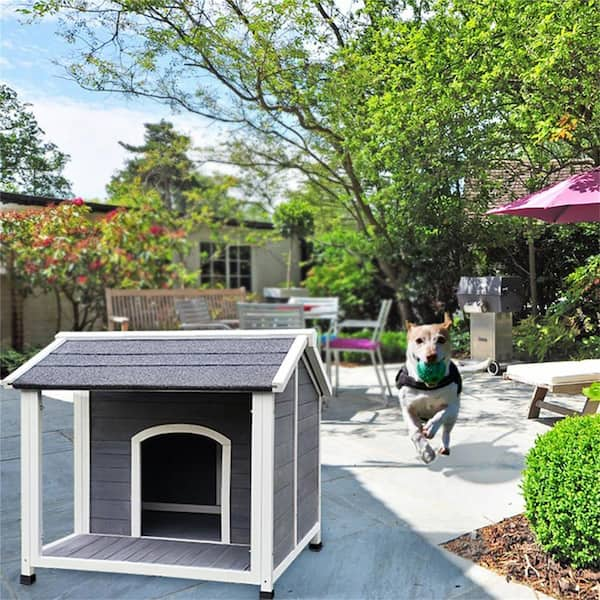In a brightly lit back garden, a small tan and white dog with a green ball featuring spots or stars in its mouth is captured mid-run, heading towards the viewer. The focus is primarily on this playful, underdog breed and a well-crafted dog kennel positioned in the bottom left of the foreground. This kennel, occupying about a quarter of the image, is elevated on white legs, constructed from dark grey wooden slats, and topped with a black tar-paper roof with white trim around its entrance. The scene is set on a stone patio that hosts the dog and its house. 

In the out-of-focus background, lush greenery and tall trees provide a summer-like ambiance, complemented by various garden furniture, including a long wooden bench, a patio table with four chairs (one sporting a red cushion), and a barbecue grill. Additionally, a vibrant pink parasol adds a pop of color, partially covering some outdoor furniture. The backdrop features a tan flat-roofed house with a large 16-paned window, a tall stone wall, and glimpses of a gazebo with a red top, further enhancing the inviting outdoor space.